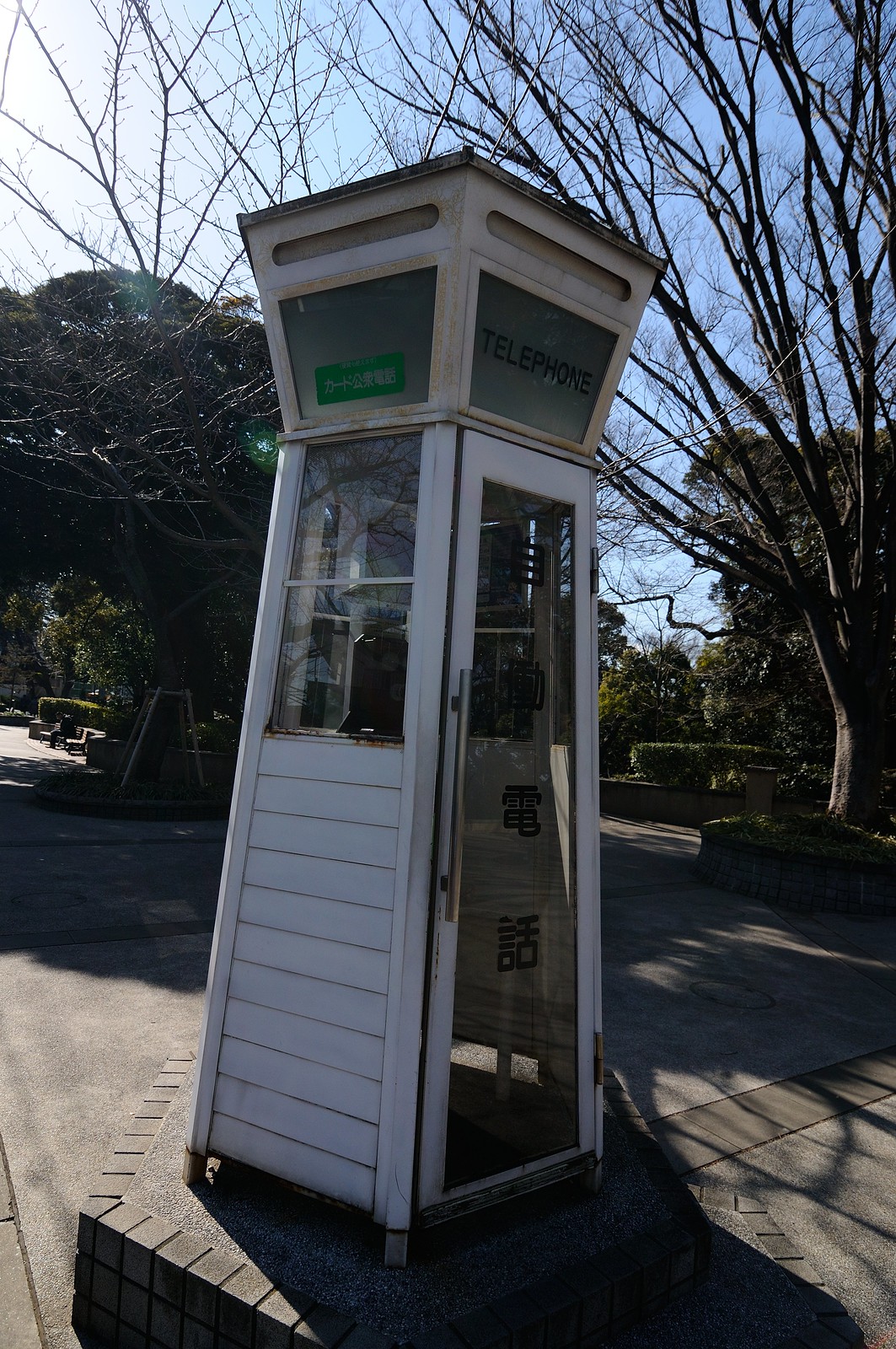This image depicts an unusual and elaborately designed telephone booth located on a raised stone platform, likely situated in a park. The distinctive structure has an obelisk-like shape that reverses itself about four-fifths of the way up, transitioning into a fluted top. Constructed as a narrow, tubular building, it features a glass door with a white border which spans the length of the enclosure. Adjacent to the door is a smaller window on the side pane, less than half the side's height, and flanked by gray panels. Etched on the glass is the word "telephone," though the enclosed area appears empty. The booth casts prominent shadows on the gray paved stone ground beneath it. The scene is framed by a deep blue sky, contrasting with dark, shadowy lines resembling tree branches. In the background, there are several trees, some with leaves and others bare, accompanied by various bushes adding to the lush park setting.